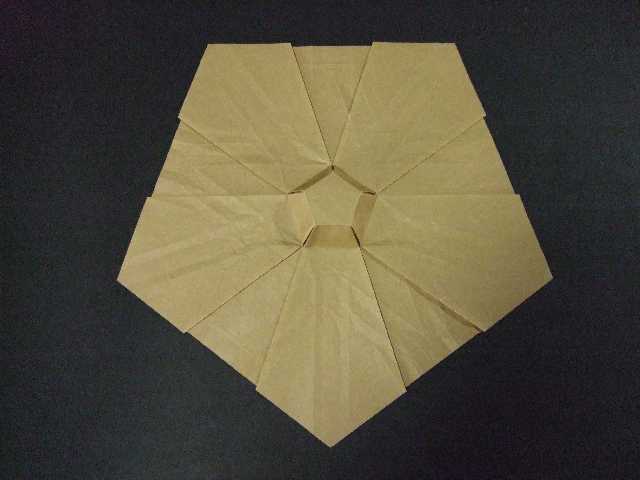The photograph features a detailed arrangement on a dark blue, possibly grainy, surface that could be a table, countertop, or carpet. The central focus is an intricate pentagon formed from overlapping brown paper napkins or similar materials. These napkins are thoughtfully arranged, resembling the structure of a house with walls and roofs, and tilted in such a way that the peak of the roof creates a triangular shape pointing towards the center of the composition. Interestingly, at the very heart of the formation lies a darker pentagon, possibly due to glue or layering, giving the whole structure an upside-down pentagon appearance. One side of the primary pentagon is flat and parallel to the bottom edge of the image, creating a striking and symmetrical visual effect.